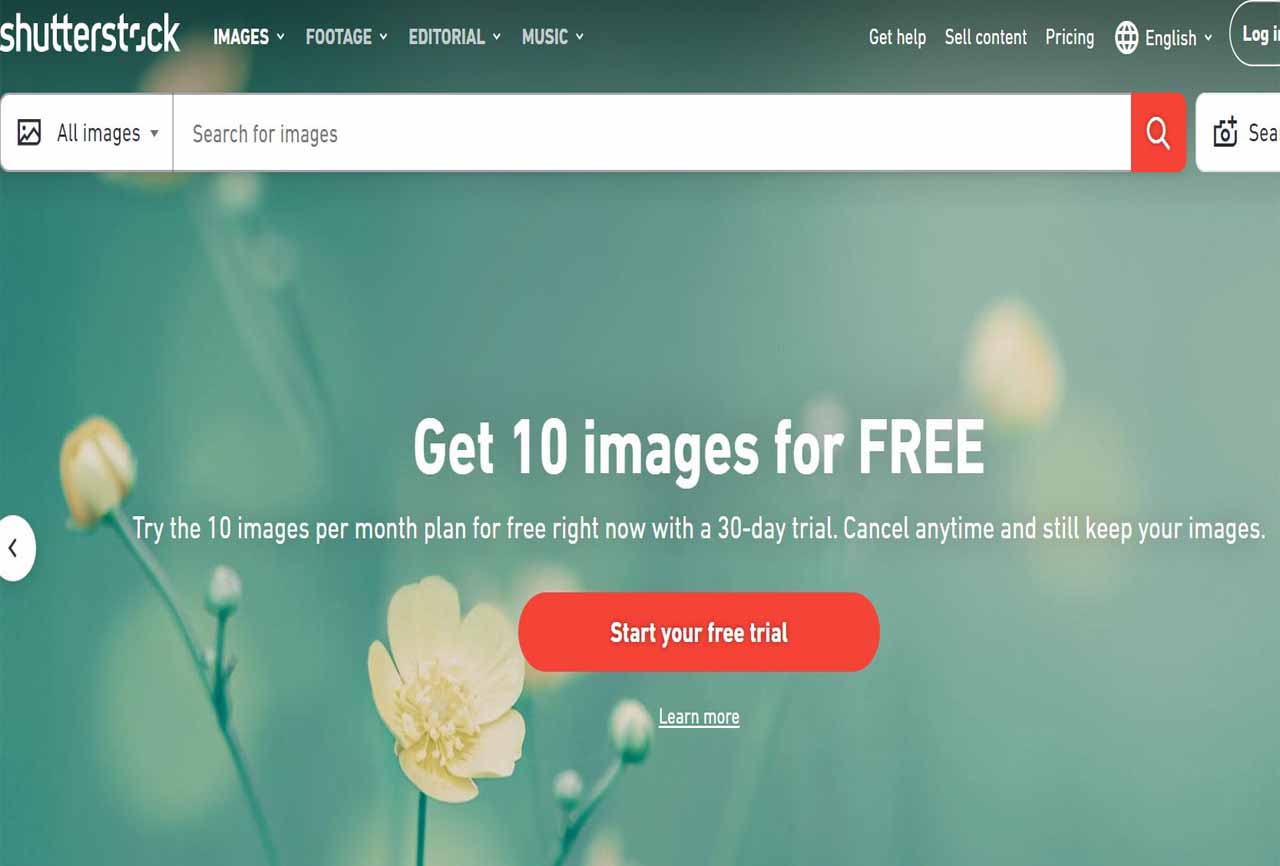This is a screenshot of a Shutterstock webpage, characterized by a green, outdoor-themed background that extends across the entire top bar and menu. In the upper left corner, the white Shutterstock logo is prominently displayed. Adjacent to the logo, the menu options "Images," "Footage," "Editorial," and "Music" are listed, each with its own drop-down menu.

The background features a nature-inspired scene with a partly opened pink flower at the left bottom section. This flower is flanked by two other buds, one on each side, that are still closed, resembling small branches or sprouts. Directly below the top menu, there's a search bar intended for image queries, with a drop-down arrow labeled "All Images" situated to the left of the search input field.